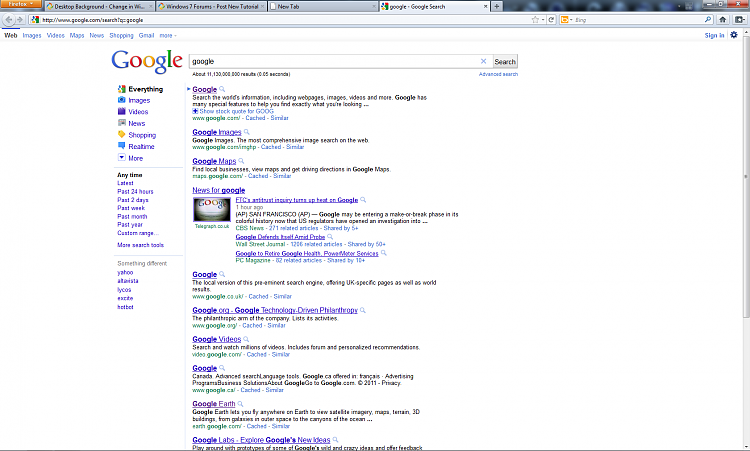This image depicts an older version of the Firefox browser interface with a distinctly retro design. In the upper left-hand corner, there's an orange button labeled "Firefox" in white text. Below this button, there are four open tabs labeled "Desktop Background," "Windows 7 Forum," "New Tab," and "Google Google Search."

The upper right-hand corner features the usual window control buttons: minimize, maximize, and a red "X" for closing the window. The address bar displays the URL "www.google.com/search?q=Google," indicating a Google search query for the term "Google."

To the right of the address bar is a Bing toolbar, along with a home icon button. Below the address bar, various search categories are listed: Web, Images, Videos, Maps, News, Shopping, Gmail, and More, with "Web" being the selected category.

The traditional Google logo appears in the upper left-hand corner of the webpage. The search query "Google" is currently entered. Down the left-hand side of the page, there are additional search filter options: Everything, Images, Video, News, Shopping, Real-time, and More, with "Everything" selected. Additional filtering options include Anytime, Latest, Past 24 Hours, Past Two Days, Past Week, Past Month, Past Year, and Custom Range.

To the right, the search results display various Google-related links: Google, Google Images, Google Maps, News for Google, Google.org, Google Technologically Driven Philanthropy, Google Videos, Google Earth, and Google Labs. The variety of vintage search engines like Yahoo, AltaVista, Lycos, Excite, and HotBot are also mentioned, adding to the nostalgic feel of the browser interface.